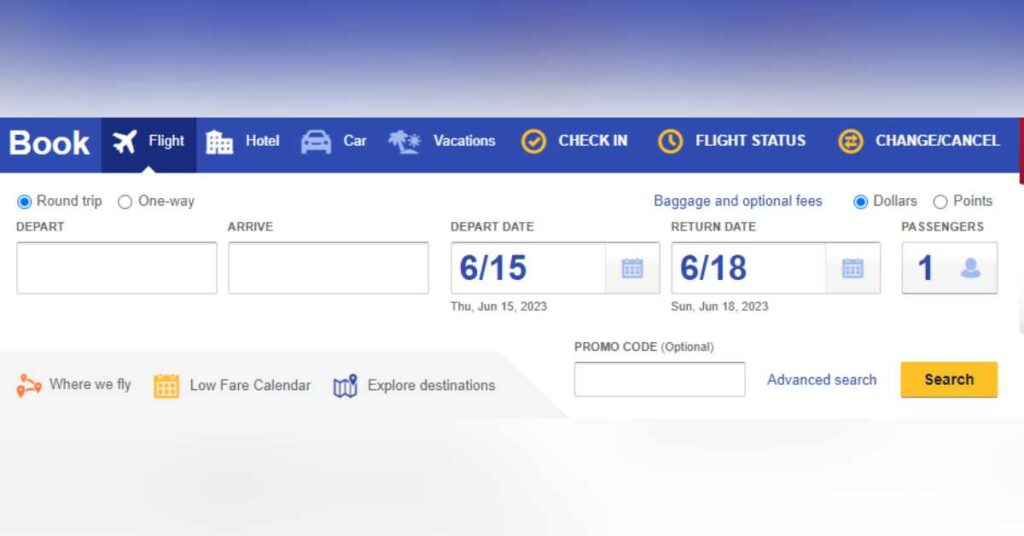The image displays a detailed booking page for a travel website. Prominently featuring a blue header at the top, the page starts with the word 'Book' in white font on the top left. Adjacent to this, there are several interactive buttons labeled 'Flight', 'Hotel', 'Car', 'Vacations', 'Check-In', 'Flight Status', and 'Change/Cancel'.

Below this header, users can choose between 'Round Trip' and 'One Way' options via easily accessible buttons. The next section includes input boxes for specifying departure time and arrival time. Continuing down, there are additional fields to enter the departure date, return date, and the number of passengers.

Further down the page, additional navigation buttons allow users to explore more options—'Where We Fly', 'Low Fare Calendar', and 'Explore Destinations'. There's a dedicated box for entering a promo code, and right next to it is an 'Advanced Search' link to refine search results. Concluding this comprehensive booking interface, a prominently placed 'Search' button invites users to initiate their travel plans.